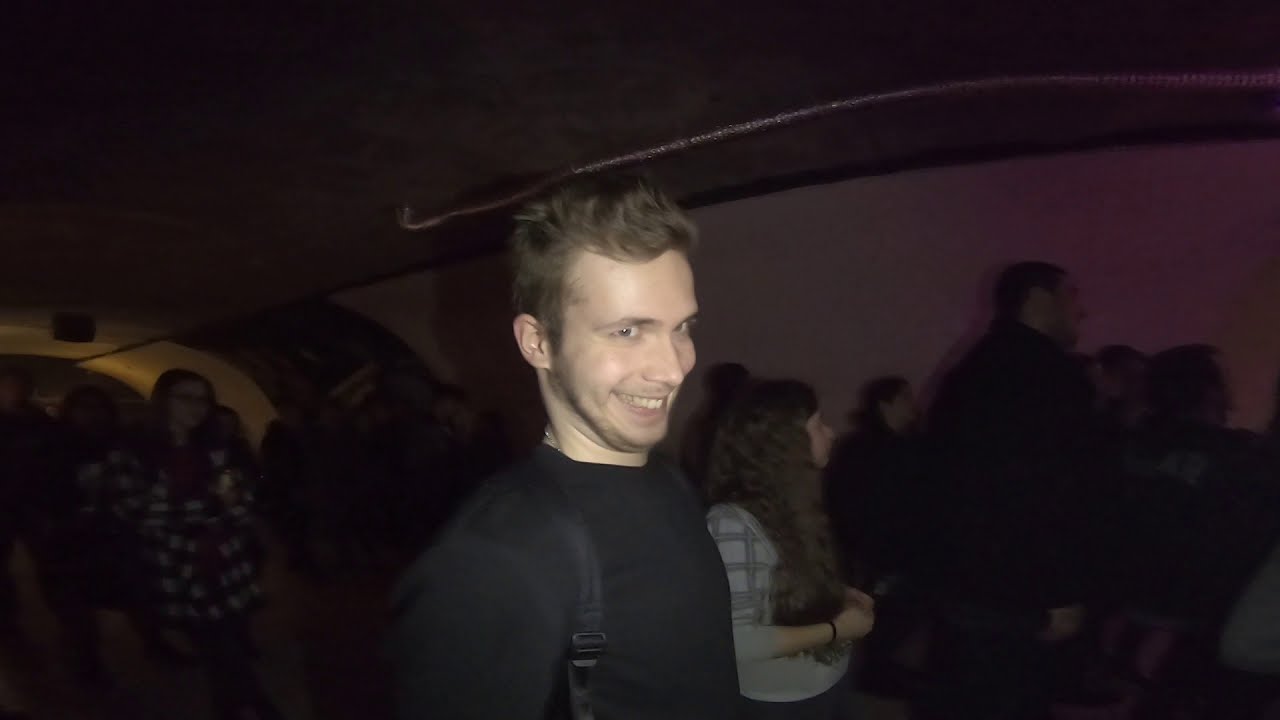In this image, a young Caucasian man with short brown hair and brown eyes is captured in a semi-dark room, possibly a club or some sort of gathering. The ambient lighting casts a purple hue across the scene, contributing to the dim atmosphere. The man, who is the central focus of the photograph, is seen from a side profile and is walking with a playful grin on his face, giving the impression he might be up to some mischief. He is dressed in a black long-sleeve shirt and has a black backpack with straps clasped around his left shoulder.

Surrounding him are numerous individuals, both males and females, who appear to be moving in the same direction, possibly through an enclosed area or tunnel. Among them is a girl with glasses wearing a black and white flannel shirt, and another with long brown hair. The walls exhibit hints of pink coloring, adding a contrasting touch to the predominantly dark setting. There seems to be a ceiling overhead with visible electrical conduits, adding to the industrial feel of the space. The scene portrays a bustling yet intimate atmosphere with roughly 15 to 20 people also captured in the background.